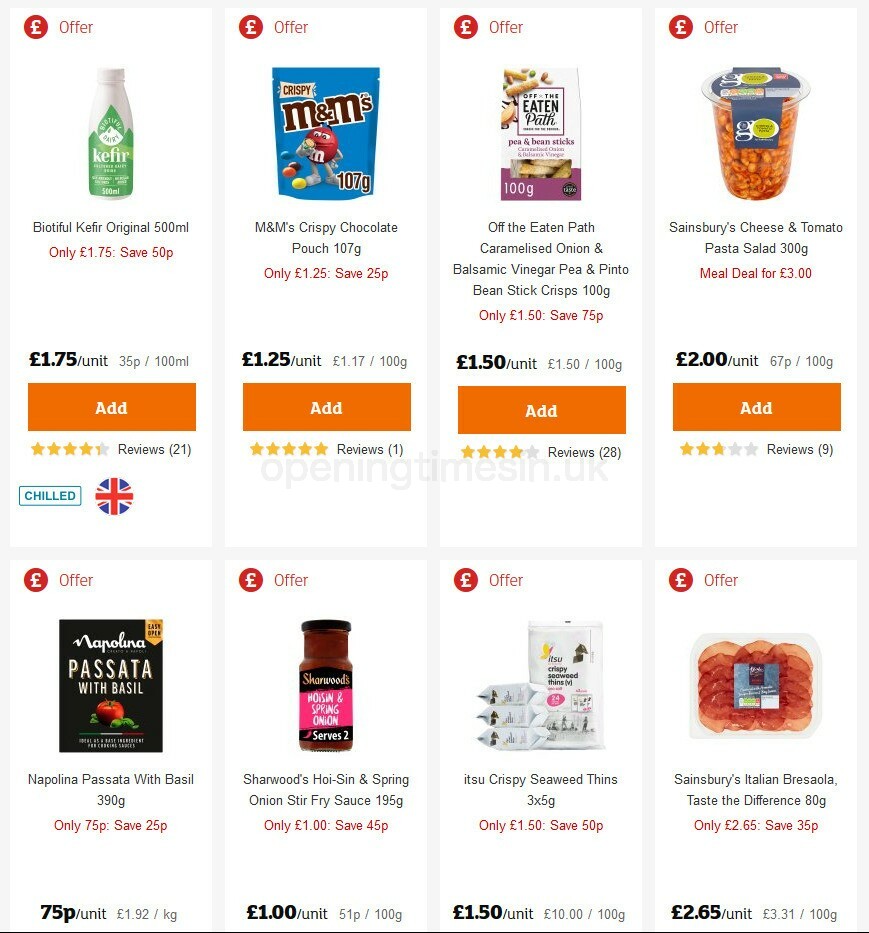This image, captured from a shopping app on a mobile device, displays eight items available for purchase in an online store, with prices listed in British pounds. The layout features two rows of products, each row containing four items. The top row items are fully visible, with clear 'Add' buttons for each product, while the bottom row is partially cut off, obscuring their 'Add' buttons.

Each product listing is encircled by a red badge indicating "Offer," highlighting their discounted prices. Every item includes a product image, a name, a brief description, and its price. Additionally, there is a note on potential savings, denoted as "Save a certain number of P," where "P" might refer to pence. 

Visible products in the top row include:

1. **Kefir** - A fermented milk drink.
2. **M&M's** - The popular chocolate candies.
3. **Balsamic Vinegar Crisps** - A unique flavor of potato crisps.
4. **Tomato Pasta Salad Cheese** - A cheese blend with tomato pasta salad.

Products in the bottom row include:

5. **Pasta with Basil** - Fresh pasta garnished with basil.
6. **Onion Fry Sauce** - A condiment designed for fried dishes.
7. **Crispy Seaweed Thins** - A healthy snack option made from seaweed.
8. **Bruschetta (Taste the Difference)** - Premium bruschetta offering from a high-quality range.

Each item's listing also includes a unit price and star-based reviews, enhancing the selection process for the shopper. Some items may have additional special messages related to promotions or product attributes.